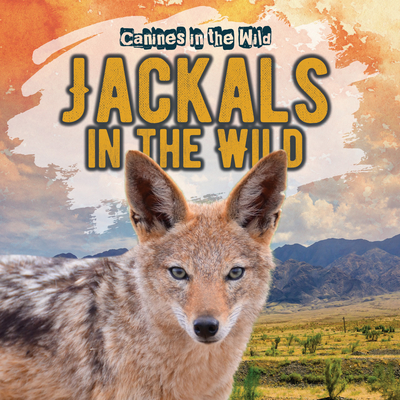The promotional artwork for "Canines in the Wild: Jackals in the Wild" is an intriguing and detailed image that prominently displays the series and episode titles in bold yellow lettering. The focus of the image is a jackal, characterized by its large ears and reddish-brown fur on its face and underside, with patches of white and dark gray fur on its back. The jackal's piercing eyes look directly at the viewer, drawing immediate attention.

Set against a nature backdrop, the jackal stands on a plane dotted with sparse grasses and shrubs. The landscape extends to reveal hills and mountains in the distance, which appear mostly bare with minimal vegetation. Above the mountainous horizon, the sky is partially blue but dominated by a thick cover of clouds that take on an orange hue towards the top, suggesting either sunrise or sunset. The overall composition conveys a wild and untamed environment, emphasizing the jackal's natural habitat. This visually captivating scene could serve as an overlay for a film, book, or magazine cover dedicated to wildlife and nature.